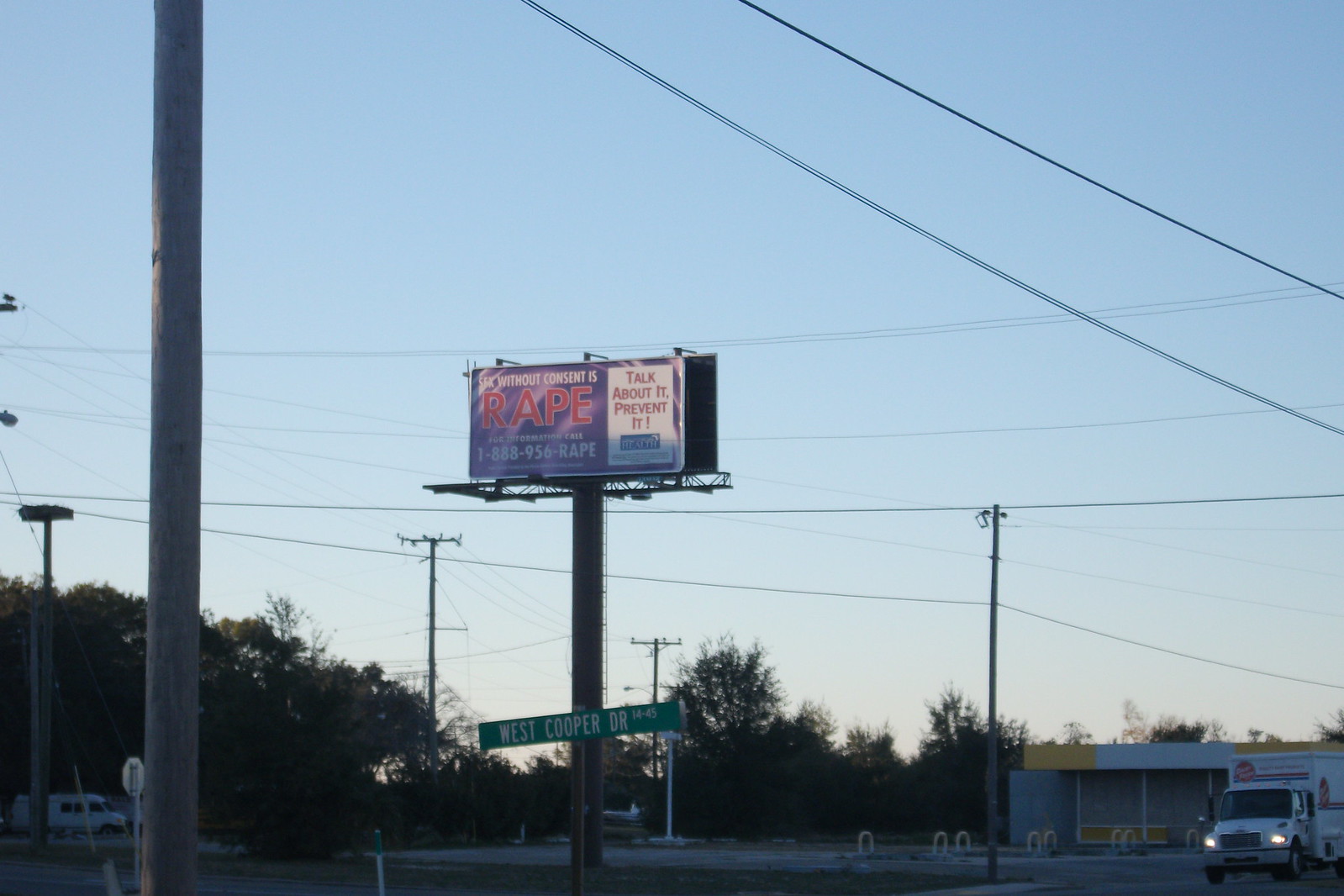The image depicts an outdoor scene along a road, with a white truck visible on the right side. In the background, there is a partially visible building, which appears to be white with yellow accents. The building has some yellow tables or similar objects in front, though the small size of the image makes it hard to discern the details clearly. 

Dominating the scene is a large billboard. The left side of the billboard has a message in red text that reads "RAPE, R-A-P-E" against a blue background, accompanied by a phone number: 1-888-956-RAPE. Below this, the text states, "Sex without consent is rape." The right side of the billboard features the message "Talk about it, prevent it" in red text against a white background. The billboard is mounted on a large stand, supported by a prominent post on the left. 

In the background, several telephone poles can be seen against a sky that, despite being blue, appears somewhat dark, possibly indicating that the photo was taken during twilight. Trees are also visible in the distance. In the center of the image, there is a green street sign that reads "West Cooper Drive."